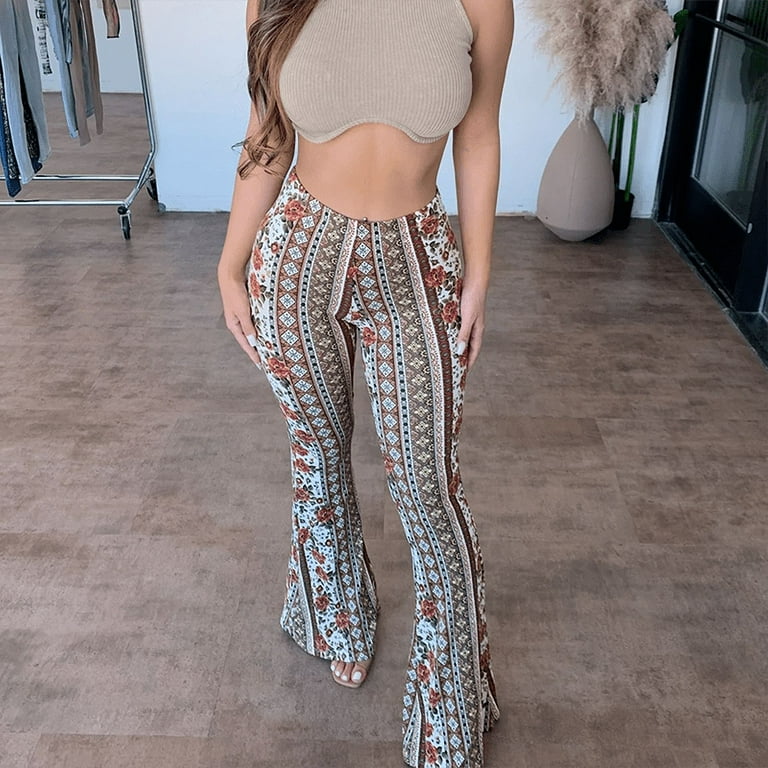This color photograph captures a woman modeling a retro-inspired outfit from the chest down to her feet. She stands in the center of the image, on a light brown floor, framed by a light blue wall in the background. To the top left, a metallic clothing rack with black caster wheels showcases a selection of gray and blue garments. To the top right, a light beige vase houses beige pampas grass, next to a black-framed window or mirror. 

The woman’s long, curly dark brown hair drapes elegantly over her left shoulder, cascading past her chest and elbows. She wears a light brown, ribbed-knit crop top that ends just below her breasts, revealing her toned midriff. Her striking patterned pants, adorned with a mix of beige, brown, cream, green, and blue colors in floral, paisley, and stripe designs, hug her hips and flare out in a classic bell-bottom style, reminiscent of the 70s. Her feet are clad in open-toe sandals, revealing perfectly manicured white toenails that match her fingernails. The woman's hands rest gently on her upper thighs, and her medium tan skin adds a warm glow to her overall look.